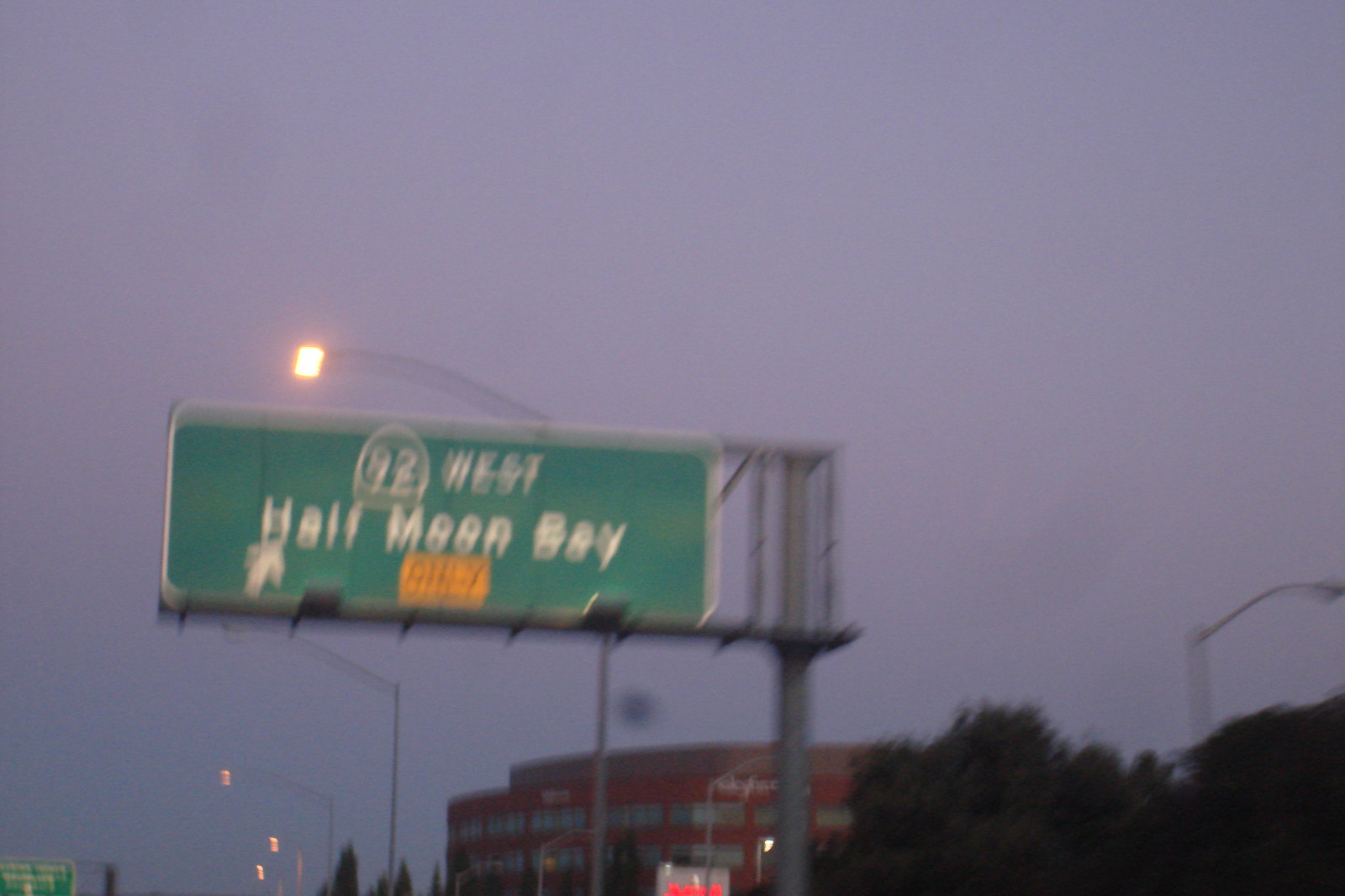This color photograph, taken from a moving car, captures a highway scene under a cloudy, overcast sky that appears purple or reddish-pink, suggesting it is either dusk or dawn. The image is notably blurry, making some details difficult to distinguish. Prominently, there is a large green interstate road sign with white text that reads "92 West Half Moon Bay" with an exit arrow pointing to the right, although smaller yellow text on the sign remains illegible. Spotlights illuminate the road sign. Below the sign, on the right-hand side of the road, there is a red-brick building with several windows, though the blurriness makes the structure indistinct. Nearby, some trees appear to be swaying in the wind. The scene is lined with highway lights, adding to the dim, atmospheric lighting of what is likely a highway exit.